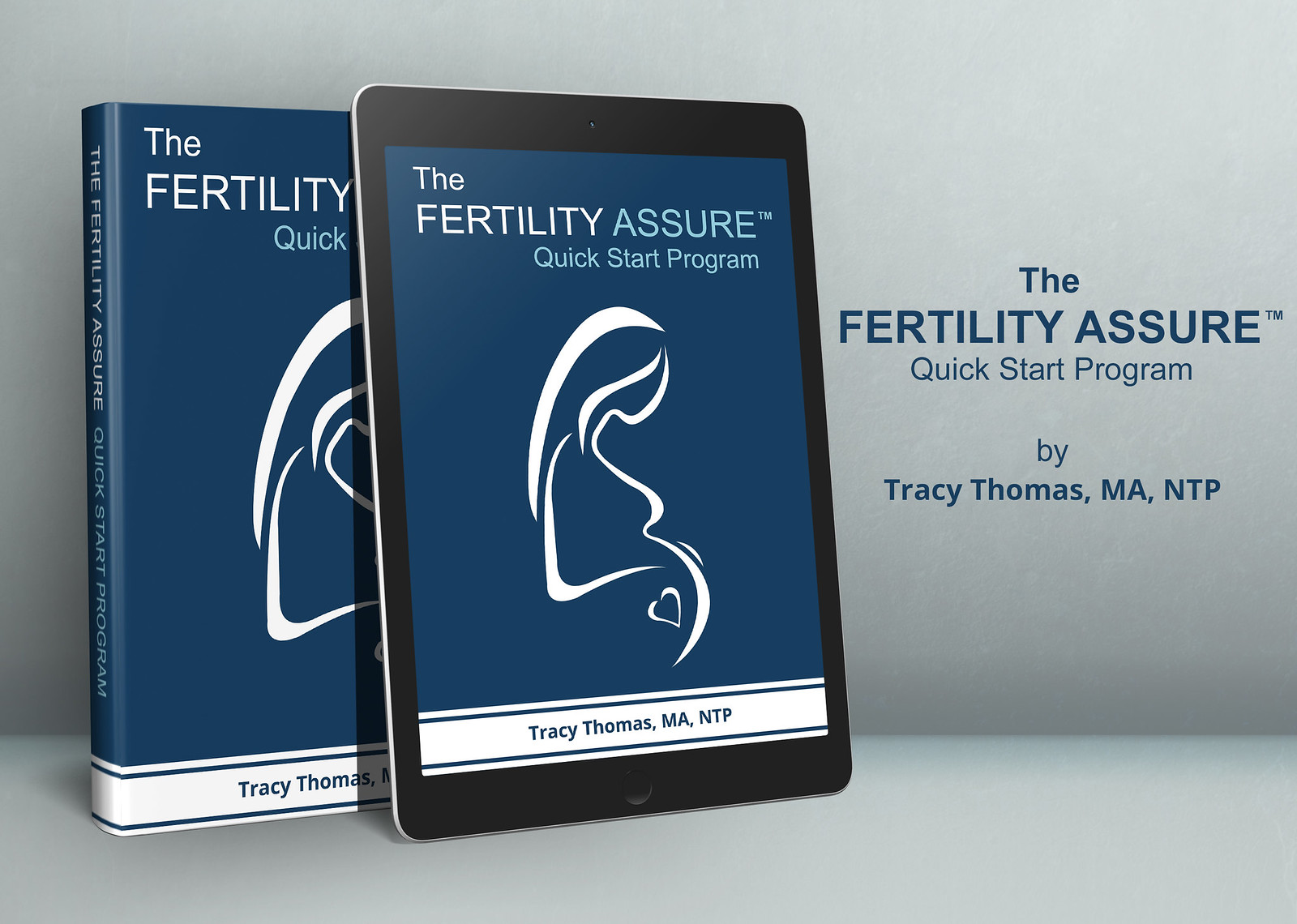The image is a detailed advertisement, likely a cover slide for a fertility program presentation, set against a gray background designed to resemble a tabletop or a wall. It features a book on the left and a tablet slightly leaning against it to the right. Both the book cover and the tablet display the same visual: a blue background with white text reading "The Fertility Assure Quick Start Program." Prominently featured in both images is an abstract logo of a side-view of a pregnant woman with a heart in her belly. The bottom of both covers has a white strip with blue text that reads "Tracy Thomas, MA, NTP." Additionally, the right-hand side of the image has blue text repeating, "The Fertility Assure Quick Start Program by Tracy Thomas, MA, NTP." This suggests the image is meant to highlight and promote the program by Tracy Thomas, potentially related to addressing fertility and possibly involving IVF treatments.